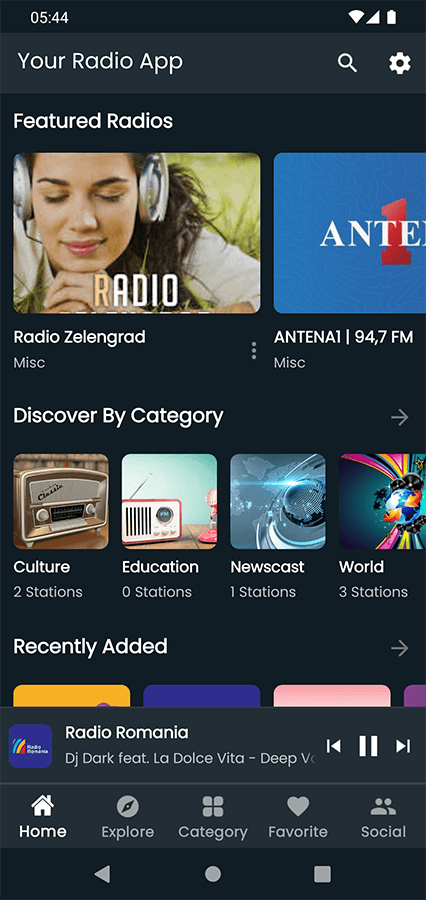The image is a vertical screenshot of a cell phone screen with a black background. At the top left of the screen, the time is displayed as "5:54." In the top right corner, icons indicate full cell signal, full wireless signal, and full battery life. Below this, a horizontal gray bar spans approximately 5% to 10% of the screen's height, displaying "Your Radio App" in text. On the right side of this bar, there is a white magnifying glass icon and a gear icon for settings.

Moving further down, the title "Featured Radios" appears in white text on the left side of the screen. Below this, two images are displayed side by side. The left image is labeled "Radio Zellengrad" and shows a young woman with headphones on, smiling with her eyes closed and her hands visible. The label "Radio" appears below her image. The right image is labeled "Antenna" (spelled A-N-T-E-N-N-1) with "94,7 FM" written vertically. The image has a blue background with partial text "A-N-T-E" and a partially cut-off "1."

Halfway down the screen, the title "Discover by Category" is visible. Below this title, four squares each display a picture and label "Culture," "Education," "Newscast," and "World." Under these labels, the text indicates the number of stations available for each category: two stations for Culture, zero stations for Education, one station for Newscast, and three stations for World.